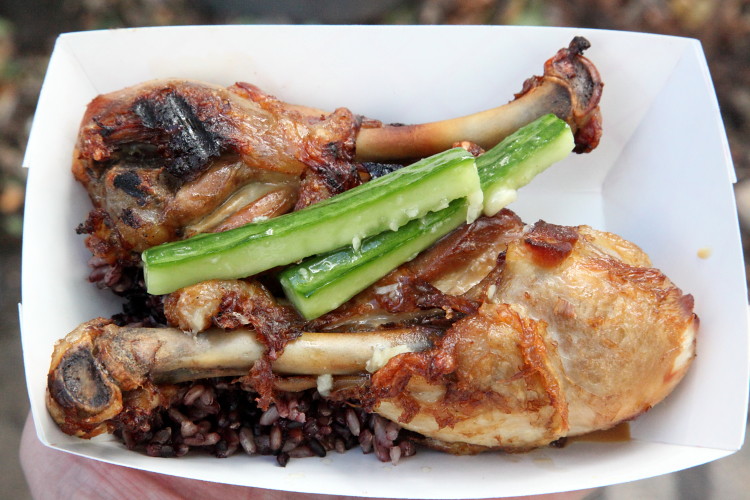The close-up color photograph captures a white paper carry-out container filled with a tantalizing meal. Inside the container are two golden-brown roasted chicken drumsticks, positioned oppositely with the top drumstick's knuckle pointing right and the bottom drumstick's knuckle pointing left. The succulent chicken pieces feature charred skin with glistening brownish sauce and sit atop a bed of dark, multi-grain rice, possibly gelatinous or basmati, adding a rich contrast in texture and color. Nestled in between the drumsticks are long, julienne strips of quick-pickled cucumber. The juice pools in the bottom right corner of the carton, hinting at the flavors saturating the dish. The blurred background, perhaps held in a caucasian hand, keeps the focus squarely on the inviting food presentation.